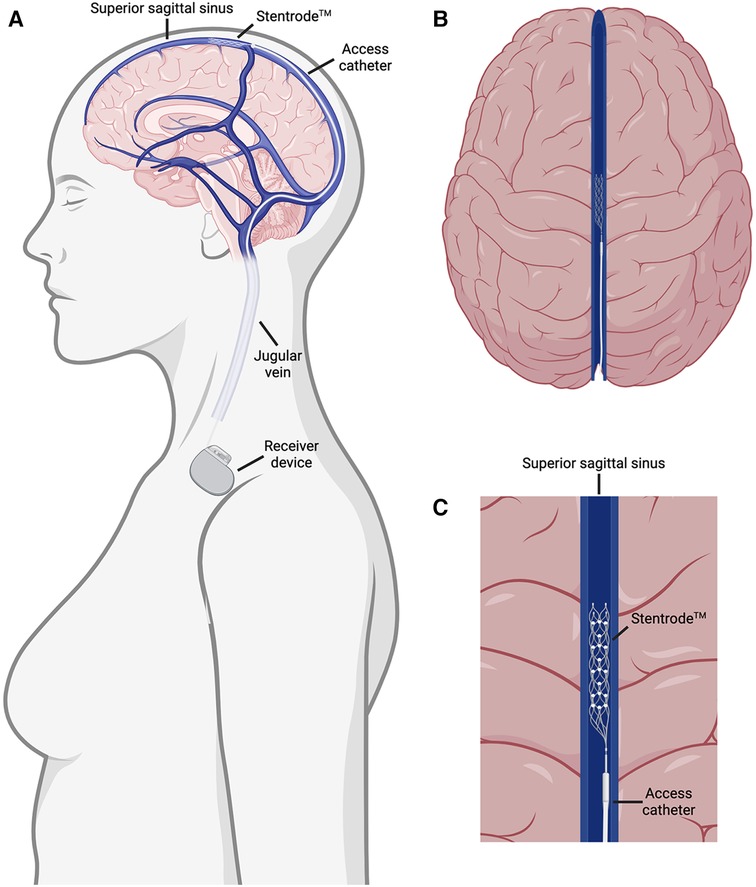This medical diagram is a detailed illustration showing three views related to a human brain and its associated vessels. The main image (labeled A) displays a minimal gray outline of the upper body of a female figure, facing left, with internal cutaways that expose key vascular details within the brain. Diagram B provides a top-down view of a drawn brain, highlighting the division between the left and right hemispheres. Diagram C zooms in on the superior sagittal sinus, illustrating the insertion point and path of a stentrode and an access catheter. The diagram includes various labels such as the superior sagittal sinus, stentrode, access catheter, jugular vein, and a receiver device, emphasizing the placement and function of the medical intervention—the stentrode—in the brain's vascular system. This comprehensive visualization aids in understanding the device's placement and the anatomical context within which it operates.